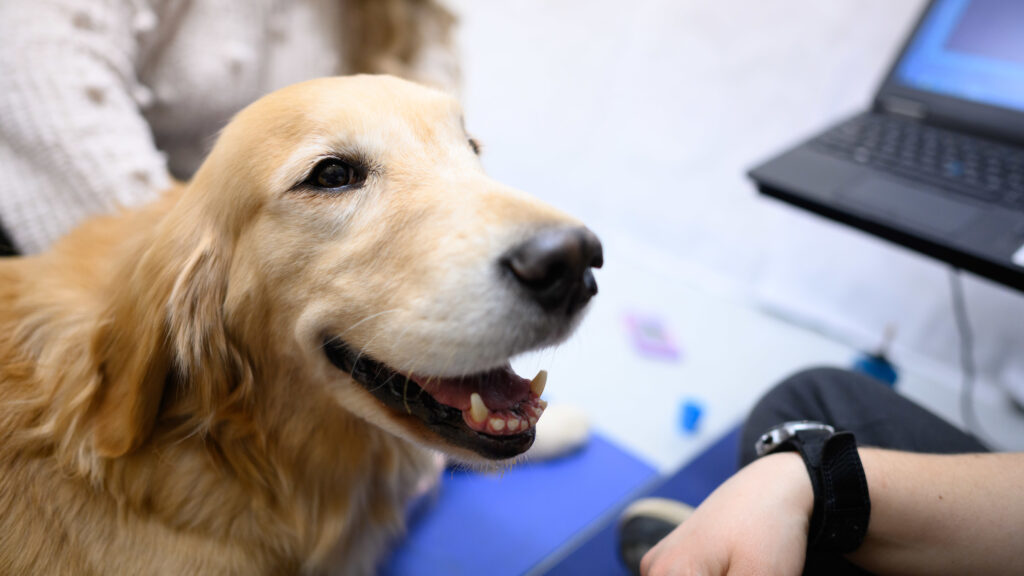The image displays a light brown Golden Retriever on the left side, with its mouth open in a way that resembles a smile, revealing some of its lower teeth including two sharp ones on each side and six smaller teeth in between. The dog has a black nose and small black eyes, with only the right eye visible. Its long, furry ear hangs down, adding to its cute appearance. The canine appears to be looking upward, possibly at its owner whose hand is visible in the lower right corner of the image. The owner, who is fair-skinned, wears a black watch with a silver dial on their right wrist. 

In the upper right corner, a black laptop sits on a white table, contributing to the office-like setting. A woman, possibly wearing a sweater, is partially visible behind the dog, with only her arm, a bit of her hair, and her upper torso, chest area, showing. The lower part of the image also features a knee, suggesting the dog is engaging with the unseen person. The background includes a section of a blue carpet, with varying shades highlighted by light patterns.